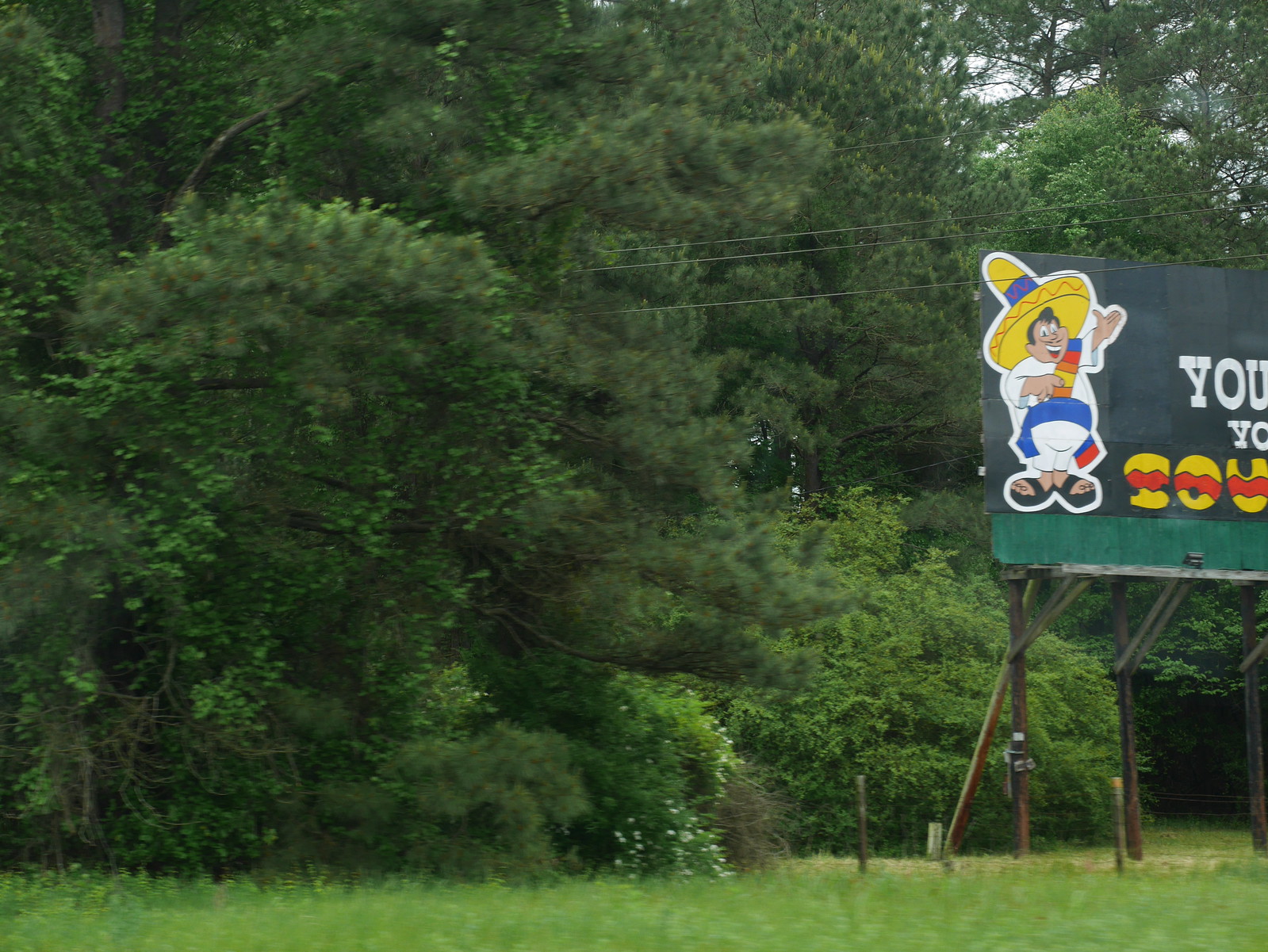The photograph captures a lush rural setting with abundant greenery and subtle wildflowers, indicative of a countryside atmosphere. A thick blanket of green grass stretches across the bottom inch of the image, while mid-frame, a slender fence supported by two brown poles marks a boundary. Looming above, three larger poles with braces support an imposing billboard, elevated about 8 to 15 feet off the ground. This billboard features a vibrant caricature of a Mexican figure, adorned in traditional attire—a large yellow hat with a blue stripe, a multicolored sash draped over one shoulder, and a blue sash around his waist. He wears white clothing and black sandals, extending his left hand in a welcoming gesture. The billboard's design includes black and green sections, with partially visible text starting with "Y-O-U" in white letters. On the opposite side of the road, the thick cluster of trees forms a dense backdrop, amplifying the rural essence of the scene. While the main focus seems to be on this roadside advertisement, subtle details such as the grayish-white flowers in the middle ground add a delicate touch to the otherwise robust and verdant landscape.